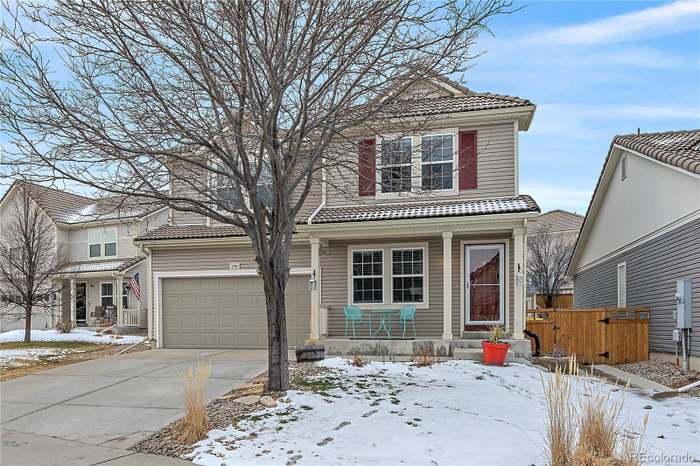In this snowy neighborhood scene, we see a central home flanked by three other houses, totaling four in the image. The main house is a tan color with a lighter tan trim and is accented by red shutters. It features a front porch adorned with two blue chairs, a glass storm door, and a distinctive wooden door. The porch also holds two potted plants—one in a vibrant red pot and another in a wooden pot. Adjacent to the driveway is a tree bare of leaves due to the winter season. To the right of the house is a wooden fence marking the backyard.

The neighboring house on the left, also tan with grayish undertones, displays an American flag on its porch. The house on the right has tile shingles and a brown gate separating it from the central home. A power box is mounted on the outer wall of this house. Scattered footprints mark the snowy ground, adding to the serene, wintry atmosphere. The sky above is cloudy, completing the tranquil yet detailed portrait of this picturesque neighborhood.